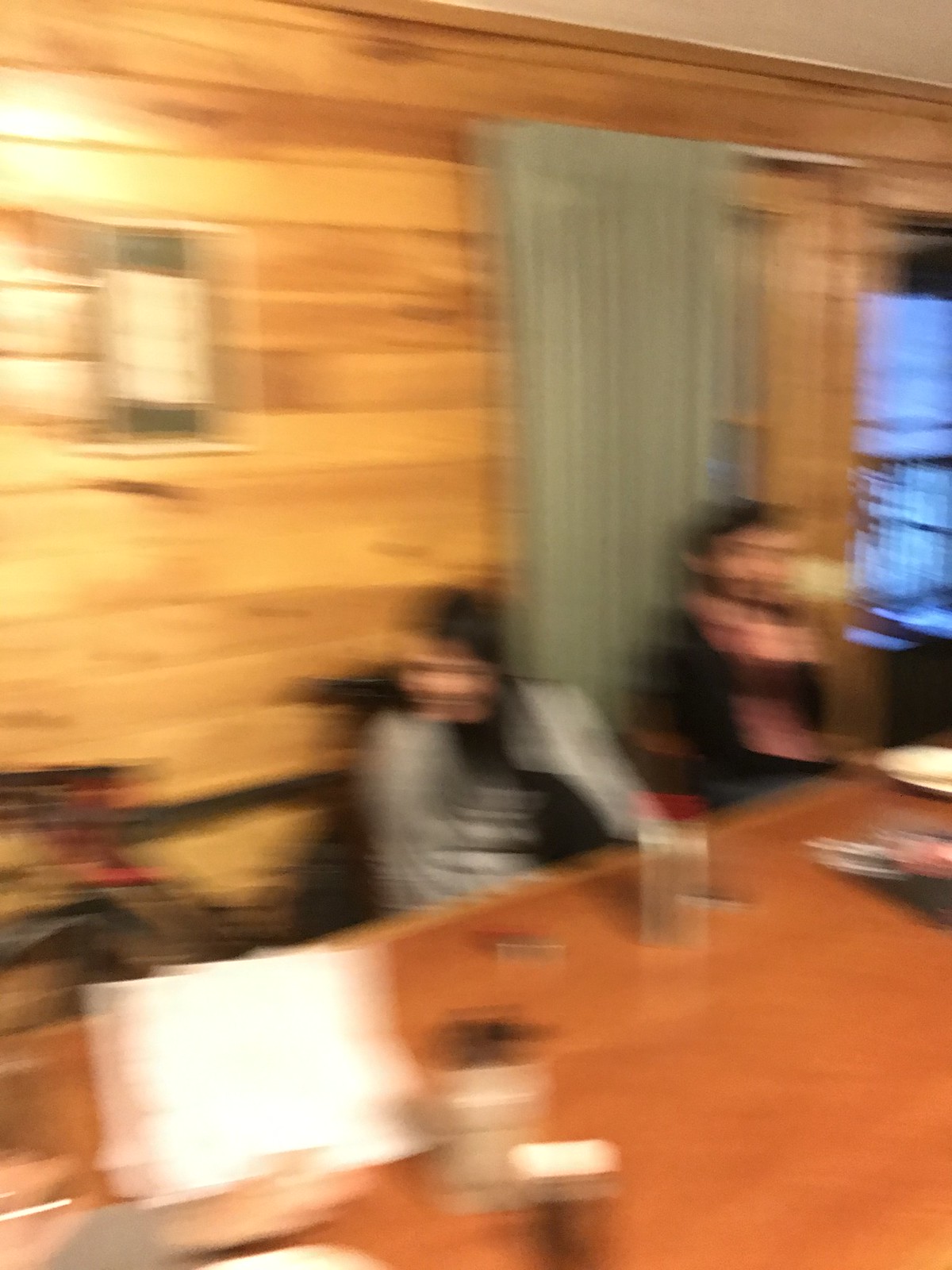This image is a blurred photograph, roughly 30% taller than it is wide, suggesting it was captured while the camera was in motion, compromising image stability. The scene is set indoors, featuring a large wooden table, medium brown in color, that occupies the bottom right corner and extends from about 20% up the left side to 40% up the right side of the image. At the table, three people can be discerned, though only two are visible. The central figure, a Caucasian female with long black hair, wears a grey sweatshirt with black arms and collar. She faces approximately seven o'clock. To her upper right is a male of similar age with short black hair in a dark shirt. 

The table itself holds several items, including papers, glasses, and plates, indicating a recently finished meal. The blurred background shows a wall made of wooden planks, partially obscured by a full pale green curtain on the right side. There is a suggestion of an open window or doorway at the very edge of the right side of the picture, with a hint of black railings and a blue-hued frame.